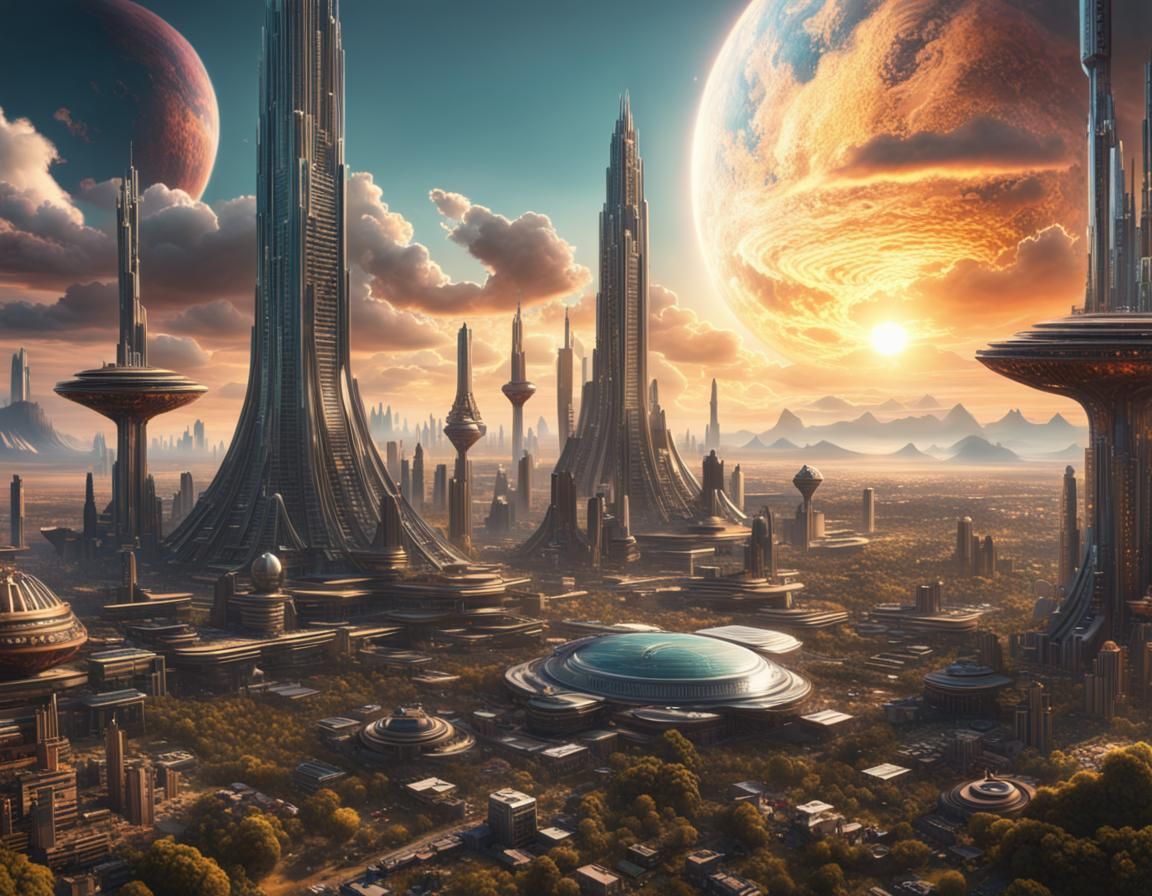This image is a highly detailed, futuristic graphical artwork depicting a vibrant and fantastical outdoor scene. Captured from an aerial perspective during the daytime, the view spans across a unique landscape filled with both natural and architectural wonders. The sky above is a solid blue, punctuated by floating patches of clouds and a bright light, possibly from the sun, illuminating the scene.

The foreground showcases a mix of curvilinear and angular structures, with numerous circular buildings scattered throughout. Prominently, at least six towering structures rise from wide bases, arching gracefully towards their narrow peaks, which ascend into tall spires that pierce the sky. Interspersed among these spires, clouds float in-between, enhancing the otherworldly ambiance. 

In the background, rolling and foggy hills provide a rugged contrast to the sleek lines of the futuristic architecture. Within this panoramic setting, two large celestial bodies dominate the upper corners of the image. On the left, a round, reddish planet almost captures the frame, while on the right, a significantly larger planet with swirling hues of yellow, gold, and blue commands attention. This larger planet, partially covered by clouds, adds a sense of depth and otherworldliness to the illustration.

The entire composition is bathed in a surreal, almost netherworld fantasy atmosphere, blending elements that evoke both science fiction and dreamy landscapes. The detailed depiction of the sky, the innovative buildings, and the planetary elements collectively create a visually arresting and imaginative scene.